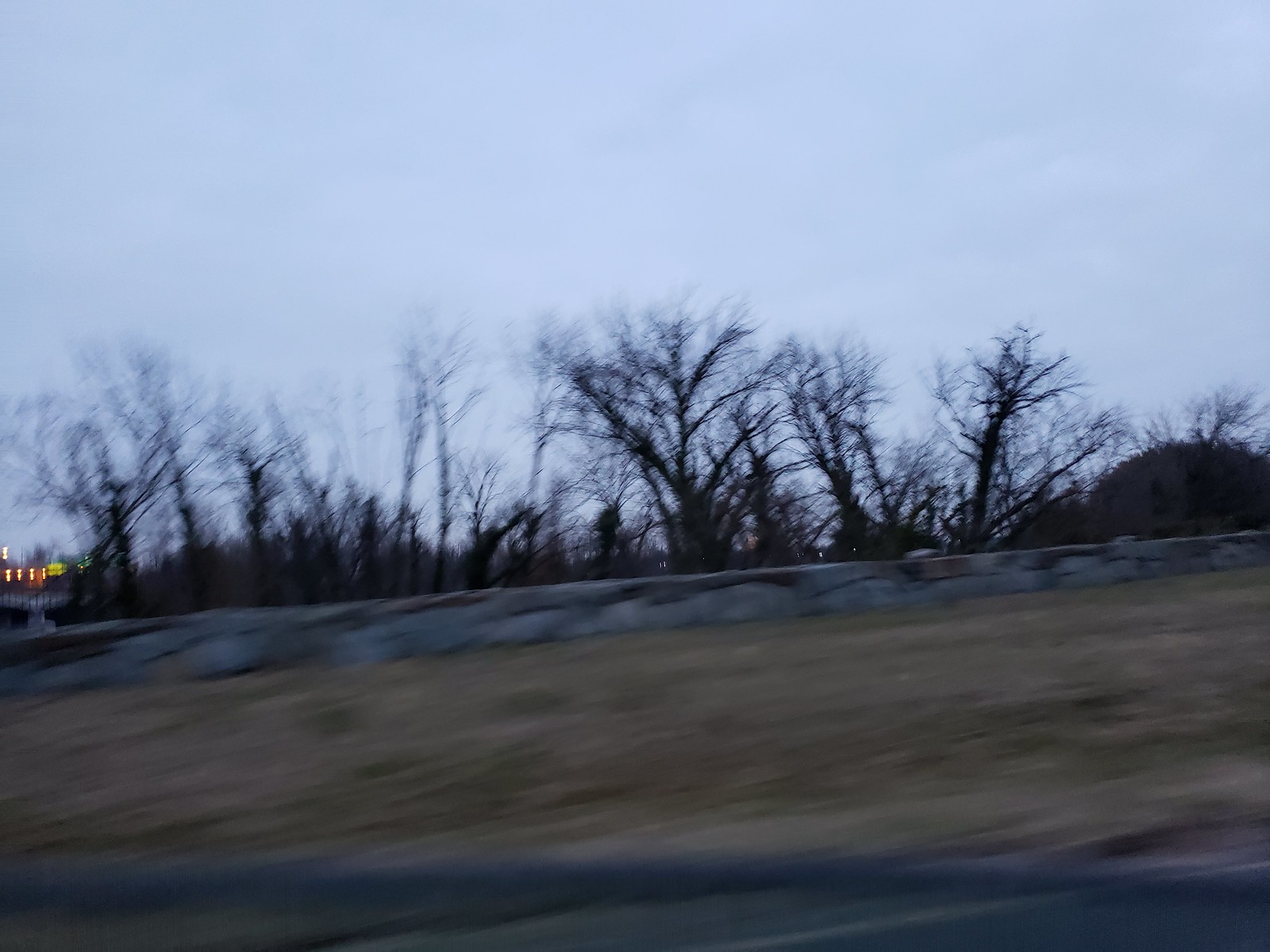The image is a blurred, digital photograph taken from a moving vehicle, possibly through a car window, capturing an overcast, cloudy day that suggests late fall or winter. Dominating the upper half is a bluish-white, fairly cloudy sky, while the background features a tree line composed of numerous leafless trees, with dark brown trunks and branches. In the middle ground, a natural stone wall runs horizontally across the scene, displaying various shades of tans and grays. Below the wall, dried grass with sporadic green patches stretches across the foreground. Additionally, a gray rope-like object is visible near the bottom. On the left side of the image, just below the center, are four or five small, indistinct orangish-yellow lights atop a small structure, possibly a drone or similar device, contributing to a mysterious element in the otherwise natural setting.